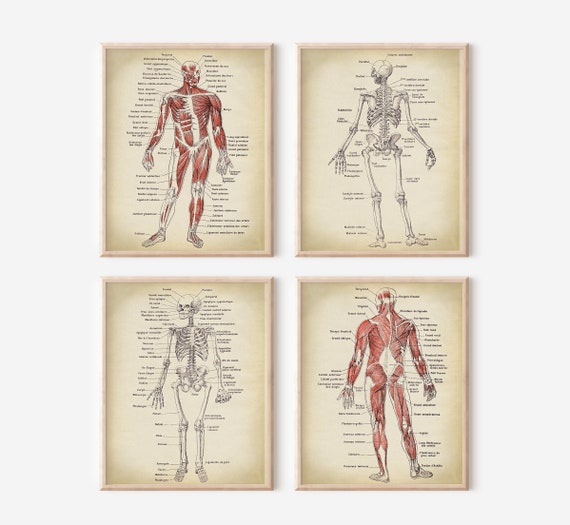The image displays a set of four framed prints, arranged in a 2x2 grid with some spacing in between, all depicting detailed illustrations of human anatomy. Each print, sourced from a vintage medical journal, is rendered on off-white, yellowed, or light peach-colored pages, giving them an antique appearance. The top left print shows an anterior view of the human muscles, highlighted in red ink, extending from head to toe with meticulous call-outs for each muscle and tendon. Diagonally across, in the bottom right corner, there's a posterior view of the same muscular illustration, similarly detailed and labeled. The top right print features the posterior view of a skeleton, depicted in meticulous black ink lines, with detailed labels identifying various bones. In the opposite bottom left corner, a front-facing skeleton mirrors the anatomical accuracy of the other, standing as a counterpart to the back-facing skeletal illustration. Together, these four prints, precisely labeled and intricately drawn, offer a comprehensive visual study of human anatomy, juxtaposing skeletal structures with muscular systems, both front and back.